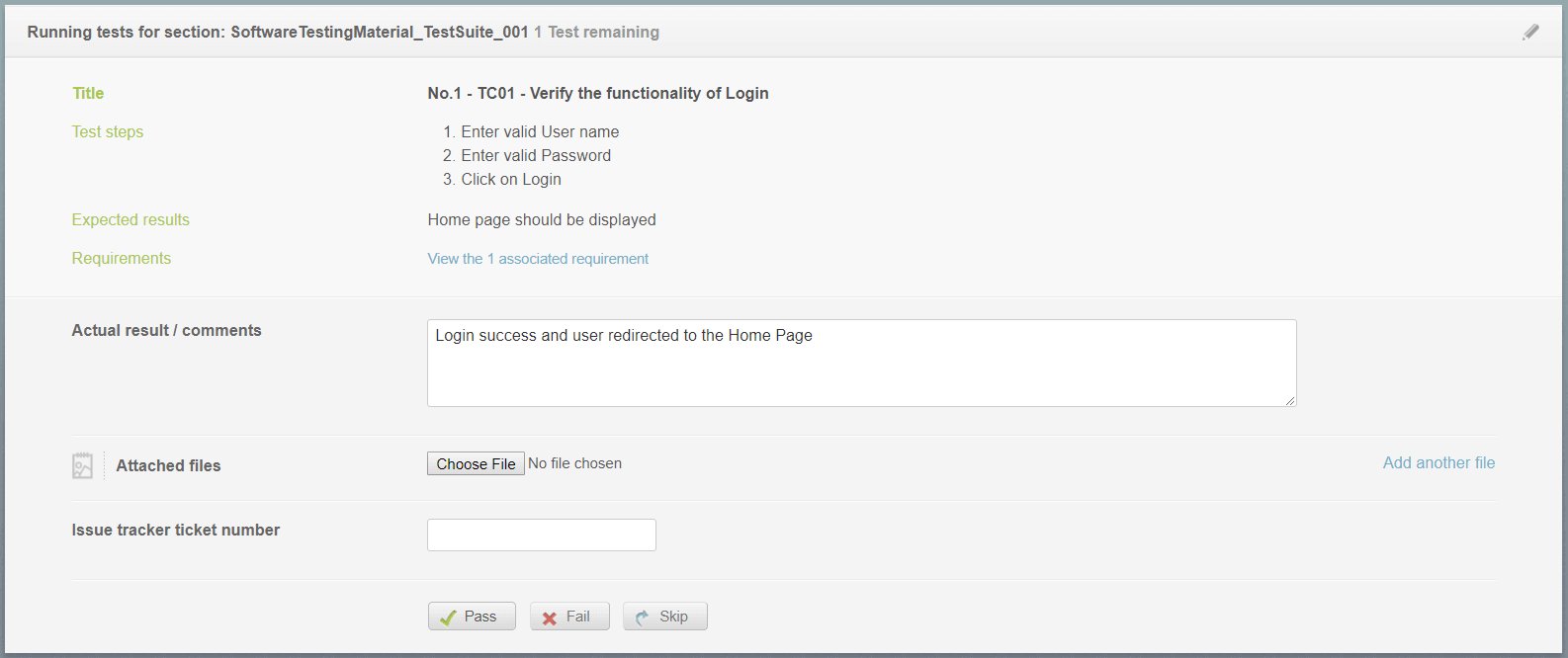Screenshot of a software testing interface, characterized by a dark green outline. At the very top, a black heading reads "Running Tests for Section: Software Testing Material Test Suite 001". Below this, in gray text, it states "1 Test Remaining". To the right, an "Edit" button is visible within the banner.

Beneath the header, in a green highlighted section, there are four listed steps: Title, Test Steps, Expected Results, and Requirements. The "Title" step is noted as "1. TC01 - Verify the Functionality of Login". The "Test Steps" include:
1. Enter valid username.
2. Enter valid password.
3. Click on login.

The "Expected Results" indicate that the home page should be displayed. The "Requirements" section prompts the user to "View the 1 associated requirement," highlighted in blue.

Following the main steps, there is a section for "Actual Results / Comments" containing a text box. The provided comment is "Login success and user redirected to the home page". Below this, there's an "Attached Files" area with a "Choose File" button, though no file has been selected. There's a field for an "Issue Tracker Ticket Number," which is currently blank.

At the bottom, three buttons are available for test result status: "Pass," "Fail," and "Skip".